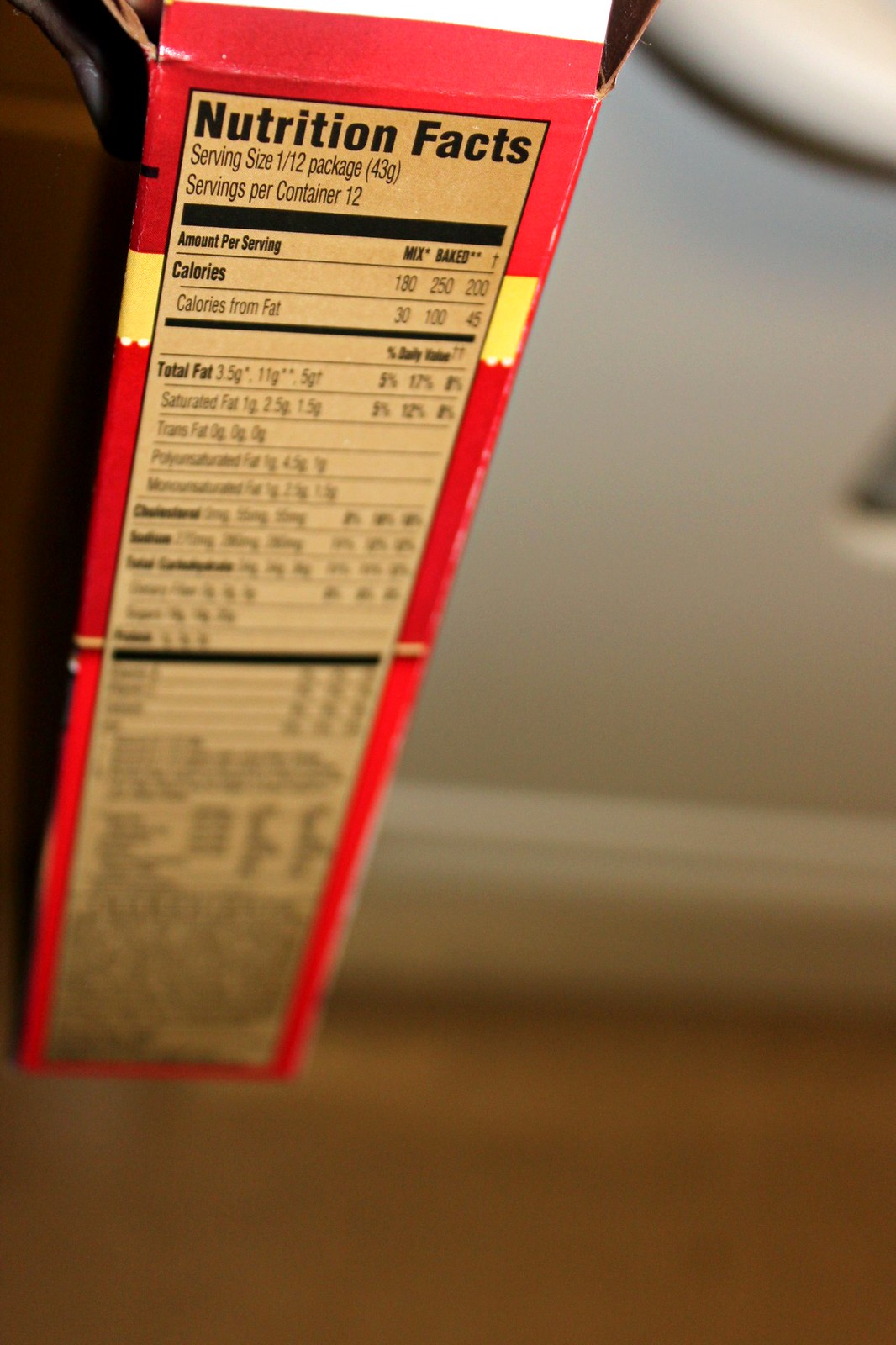On a vibrant red box, a detailed white nutrition label provides comprehensive information about the product's nutritional content. The top section prominently displays "Nutrition Facts" and lists the serving size as one-twelfth of the package (43 grams), with 12 servings per container. It details the calorie content, indicating 180 calories per serving in its mix form and 250 calories when baked, with an additional 200 calorie value suggesting an alternative nutritional breakdown.

The label meticulously itemizes the fat content, including total fat with its breakdown into saturated fat, trans fat, polyunsaturated fat, and monounsaturated fat, each accompanied by both gram quantities and daily value percentages. Further down, it mentions cholesterol, sodium, total carbohydrates, and protein, although these figures are less legible and slightly blurred. Overall, the label presents an in-depth and specific nutritional analysis, helping consumers make informed dietary decisions.